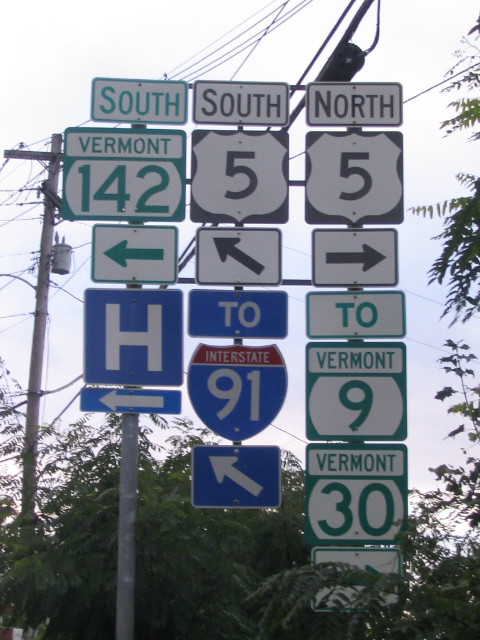The photograph captures a dense cluster of street signs on a single silver metal pole against the backdrop of green bushes, trees, and a large electric pole with a silver transformer. Prominently featuring Vermont's road signage, the topmost sign is green with white text, reading "South Vermont 142" and includes a directional arrow pointing left. Directly below it, a blue and white hospital sign with a large "H" indicates a left turn. Centrally located among the signs is a black and white "South 5" sign with an arrow pointing diagonally left. Beneath this is an Interstate shield sign in red, white, and blue, marked "2 Interstate 91" with an upward-pointing arrow aiming slightly left. To the right of these, there's a "North 5" sign. Additionally, at the bottom right, a green and white sign points right towards "2 Vermont 9" and "Vermont 30." Telephone lines traverse the upper part of the image, enhancing the urban intersection ambiance.